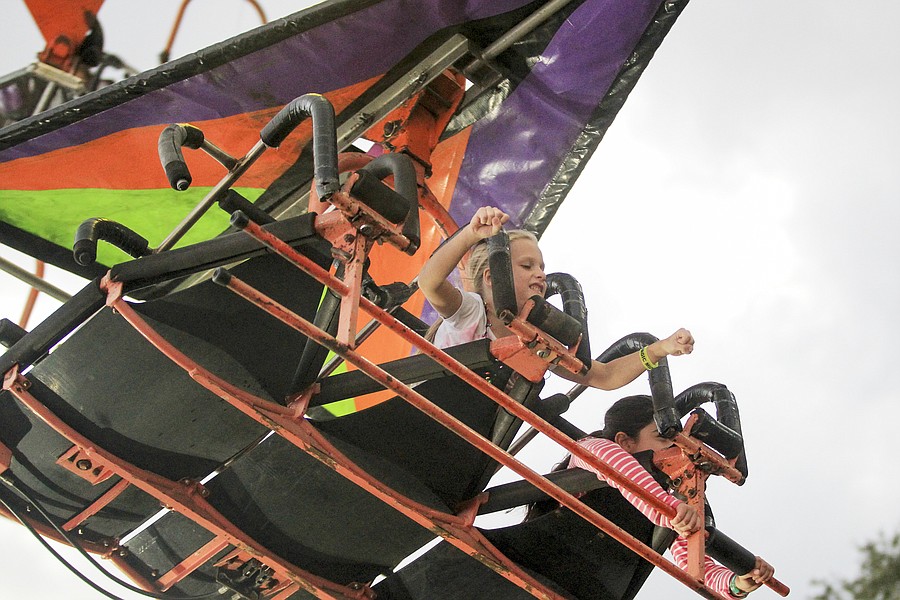This image showcases an amusement park ride on a cloudy day, with a parasailing-like glider system that features a large triangle-shaped canopy made of purple, red, and lime green fabric. The glider is supported by a robust metal bracket system that suspends three padded sleds equipped with safety harnesses and handles. The sled on the left is empty, while the central sled supports a blonde-haired girl wearing a short-sleeved shirt and a payment-indicating bracelet. She is gripping the handles, projecting a sense of apprehension, with her hands fisted in the air. To her right, a shorter brunette girl in a long-sleeved pink and white striped top enjoys the ride with her arms raised confidently. Her sled sits slightly back, as her head doesn't reach the end of the padded seat. The ride is elevated high enough to show the tops of some trees beneath the cloudy sky, underscoring the thrill and height of the overall experience.